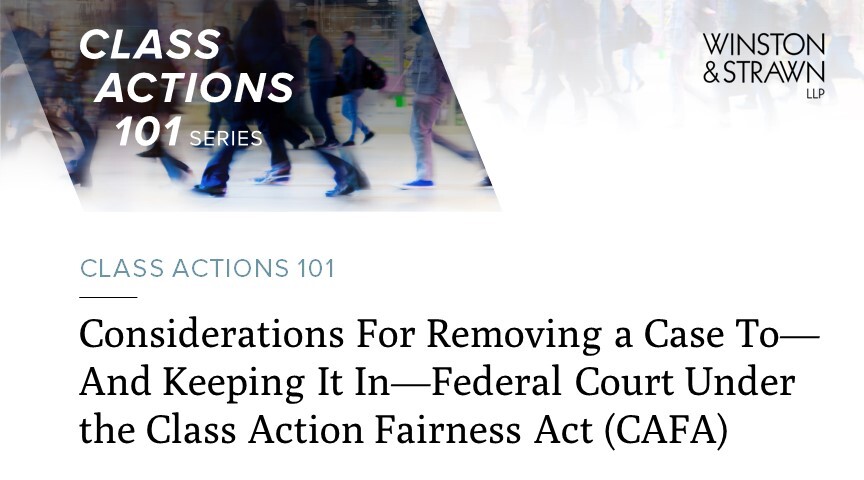**Image Caption:**

The image is a left-to-right horizontal layout depicting what seems to be the preview of an online article, likely viewed on a computer or smartphone. The background is a plain white, akin to a computer screen's default color. At the top of the image, slightly out of focus and blurred, are people walking, which serves as an indistinct background. Bold white text reading "Class Actions 101" is prominently displayed over this scene, with a less bold subtitle also in white.

On the right side, the same image of walking people appears again but with a white overlay, making the figures less visible. Over this overlay, in black text, it reads "Winston Strong LLP." 

Below this, on the left-hand side against the white background, the title "Class Actions 101" is repeated in bold black text with a small black underline beneath the word "Class." The main heading is also bold and black, with the first letter of each significant word capitalized: "Considerations for Removing a Case and Keeping it in Federal Court under the Class Action Fairness Act (CAFA)."